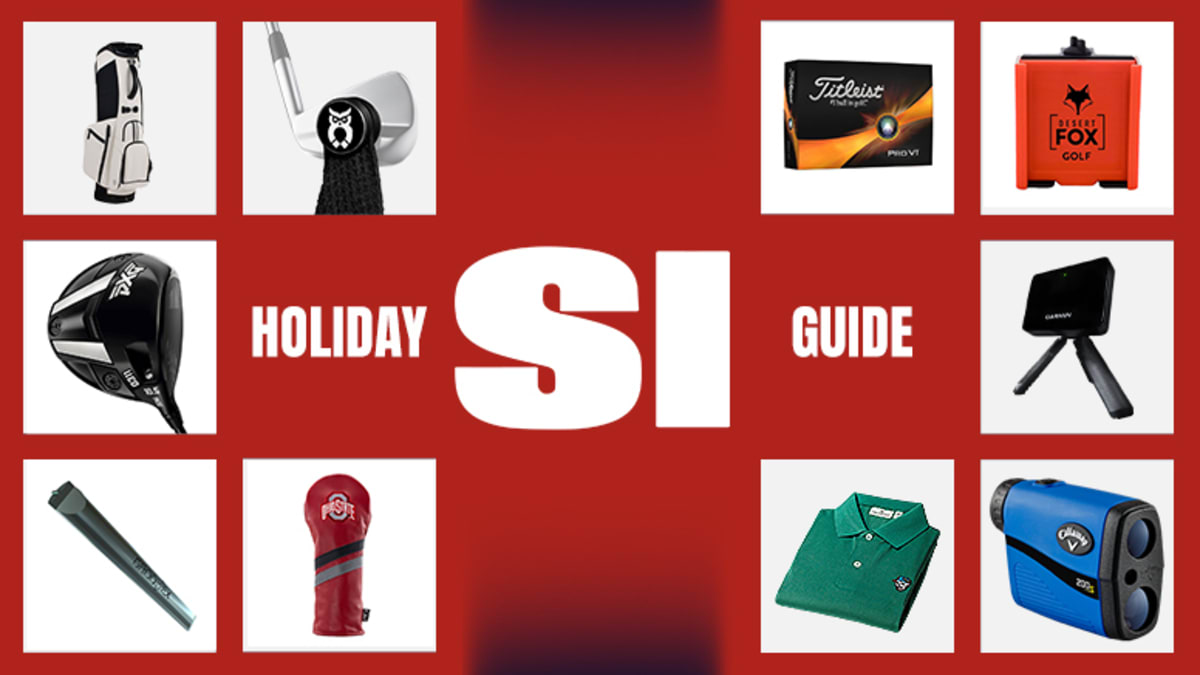The digital poster features a striking red background adorned with a collection of 10 neatly arranged square-shaped images, each set against a white backdrop. Five images are positioned on the left, mirrored by five on the right, creating a balanced design. The central focus of the poster is the bold, capitalized white text reading "HOLIDAY SI GUIDE," which spans horizontally across the middle of the layout.

On the left side, the topmost image showcases a golf bag, followed by a single golf club. The middle row presents a close-up shot of another golf club. Below that, there is a green, elongated item, possibly a golf sock. The bottom-most image may represent a cylindrical or red item, which could be interpreted as a piece of boxing equipment.

The right side starts with an image of a box labeled "Titleist Pro 4," succeeded by another box with "Fox Golf" inscribed on it. The middle row reveals a tripod stand, then a green t-shirt appears in the row below. Finally, the bottom image features binoculars.

Overall, the poster radiates a holiday vibe with its vivid red background and white accents, visually supported by an assortment of gadgets and sports gear neatly encased within white squares.